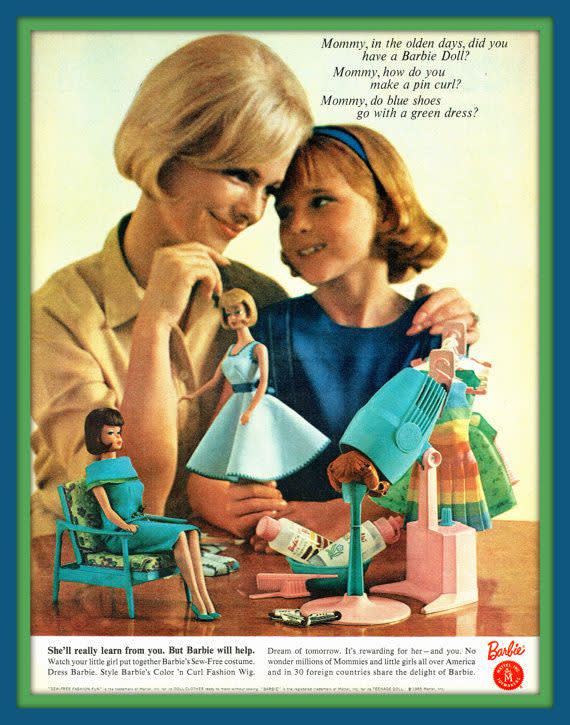This vintage advertisement for Barbie dolls, possibly featured in a parent-focused magazine, presents a tender scene of a mother and her daughter bonding over their love for Barbie. Set against a blue and green bordered background, the mother, dressed in a cream-yellow buttoned shirt with a collar and sporting a short blonde haircut with bangs, lovingly presses her forehead against her daughter's head. The young girl, with reddish-blonde hair held back by a blue hairband, is wearing a blue dress as she holds a Barbie doll in her right hand. 

In front of them on a wooden table is an array of Barbie accessories, evoking a beauty salon setting: a dark-haired Barbie seated in a chair, a blue-green blow dryer on a pink pedestal, and several small bottles possibly containing shampoo, along with a comb, a brush, and what appears to be a hair curler. 

The upper right corner of the advertisement features childlike queries in black cursive: "Mommy, in the olden days did you have a Barbie doll? Mommy, how do you make a pin curl? Mommy, do blue shoes go with a green dress?" At the bottom of the ad, a tagline reads, "She'll really learn from you but Barbie will help," followed by additional text and a distinctive round red Barbie logo in the bottom right corner.